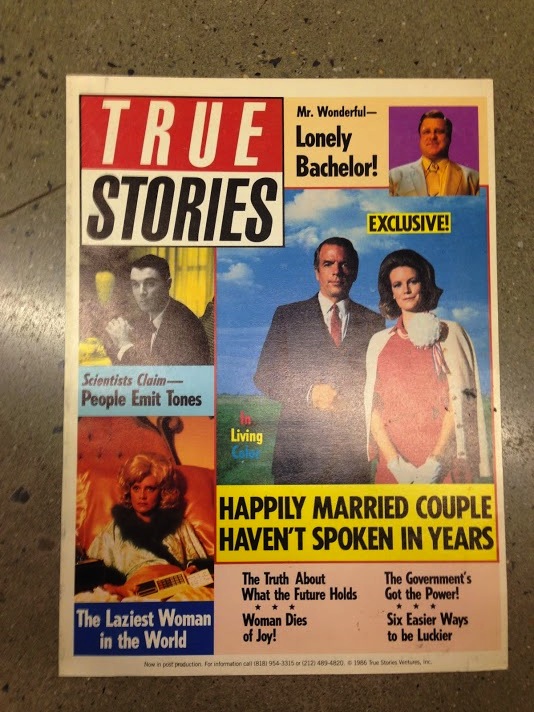The image is a vertically aligned, rectangular photograph showcasing the cover of an older tabloid magazine titled "TRUE STORIES." The background of the image appears to be a brown and black speckled tile surface, highlighted by a visible grout line in the upper left corner.

The magazine cover features a prominent title in the upper left-hand corner, with "TRUE" in large white caps and "STORIES" in large black caps, surrounded by a black border. To the right of the title, bold text reads "MR. WONDERFUL...," followed by "LONELY BACHELOR!" beneath it, depicting a man wearing a yellow shirt and a light-colored suit jacket. Below this, the word "EXCLUSIVE!" introduces a picture of a man and a woman sitting next to each other, captioned "HAPPILY MARRIED COUPLE HAVEN'T SPOKEN IN YEARS" in capitalized black letters against a yellow background.

On the left side of the cover, under the "TRUE STORIES" title, there's another picture of a man in a suit with the text "SCIENTISTS CLAIM PEOPLE EMIT TONES." Below this, an image of a woman is labeled "THE LAZIEST WOMAN IN THE WORLD." At the bottom, smaller black text states "THE TRUTH ABOUT WHAT THE FUTURE HOLDS," followed by three stars, and then "WOMAN DIES OF JOY." To the right of this, it reads "THE GOVERNMENT GOT THE POWER," followed by three more stars, and then "SIX EASIER WAYS TO BE LUCKIER." 

The cover also features a vintage aesthetic, with a woman wearing white gloves, a sweater from the 1950s, and poofed-out hair, while a man is depicted in a black suit with a red tie, echoing the classic styles of the era.